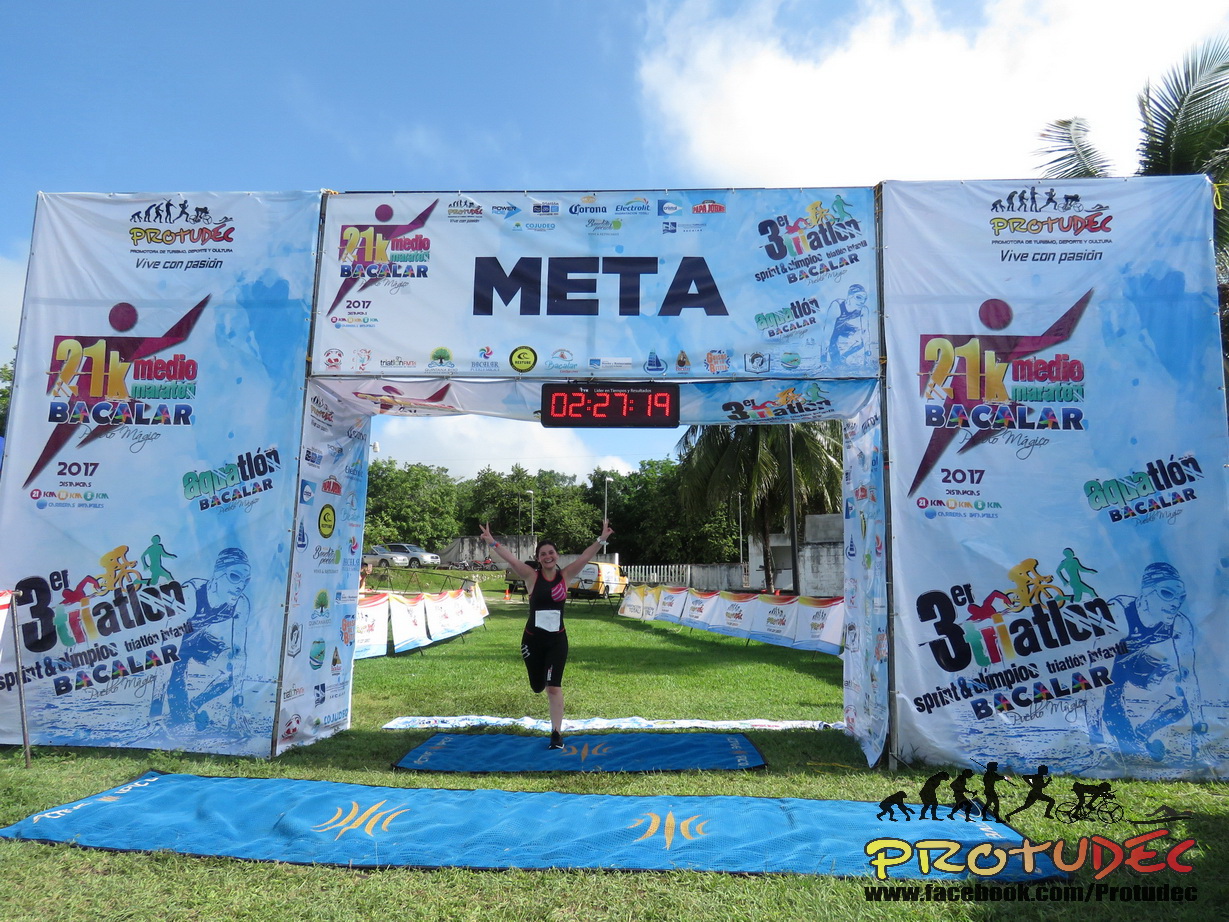The image captures the finish line of a triathlon event on a grassy field during midday. The top portion of the image features a clear blue sky with a few puffy white clouds and some palm tree branches on the right. Dominating the middle section is a large archway structure marking the finish line, featuring several banners. The banners display various sponsor names such as Meteo, Bacalar, Protudec, Corona, and Papa John's, along with event details like "21K" and "2017 3 Triathlon." A digital timer above the archway reads 02:27:19 in red.

In the center, a jubilant female runner wearing black bike shorts and a black tank top is seen crossing the finish line with her arms raised in a peace sign. Her face glows with a huge smile. The ground beneath is covered with blue rugs or towels adorned with gold decorations, and the area is lined with white signs and blue barriers. Further back, the background shows additional green trees, some traffic cones, guardrails, a distant fence, and some parked cars, all under a vibrant daytime sky.